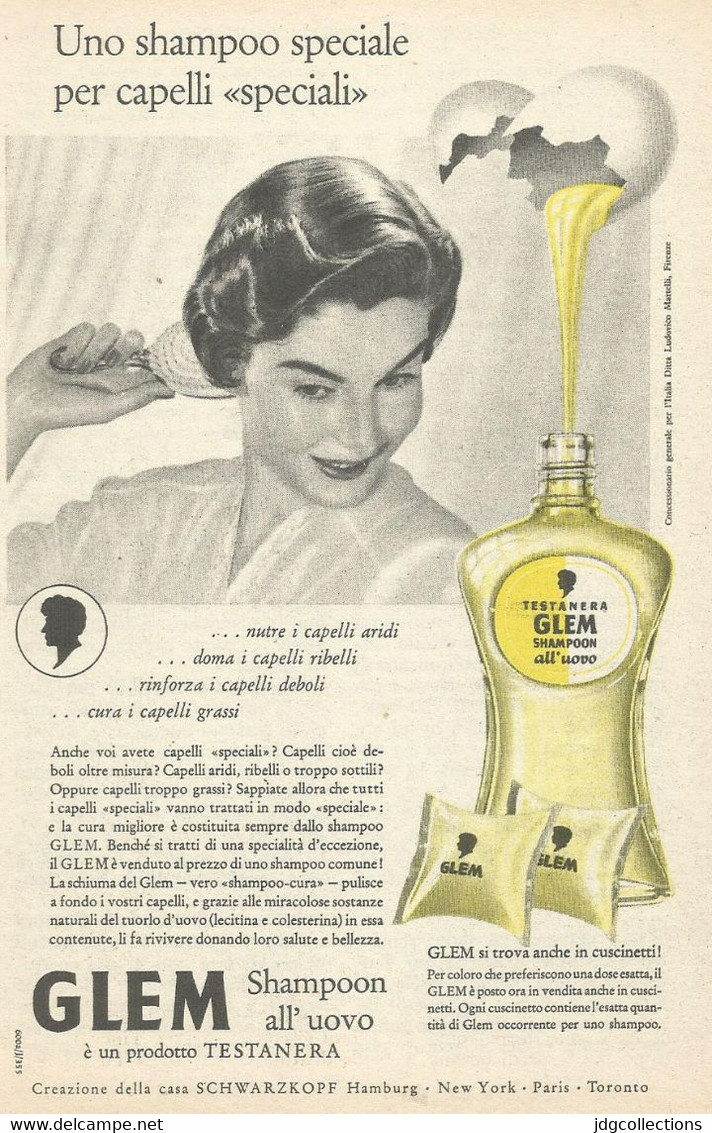The image is a vertically oriented, antique newspaper advertisement for a shampoo, appearing in either Italian or Spanish, printed on faded, yellowed paper reminiscent of the 1920s to 1950s era. In black and white, the main visual features a woman with short hair combing it with her right hand, her head tilted slightly downward while looking directly into the picture. She is captured from the shoulders up, exuding a classic elegance with visible lipstick despite the monochrome. To the right of the woman is a noteworthy cracked egg, pouring its yolk into a stylized, glass shampoo bottle below, which is distinctly colored in yellow and gold amidst the rest of the black and white ad. The bottle prominently displays the word "GLAM" and hints at the use of egg in the shampoo formulation. The ad is laden with text, primarily in a foreign language, with phrases like "UNO SHAMPOO SPEZIALE PER CAPELLI" at the top and "GLAM SHAMPOO AL UOVO" in bold at the bottom. The overall composition suggests the ad is an old-school promotion for a specialized egg-based shampoo, with additional context provided by the website www.delcampe.net at the bottom.